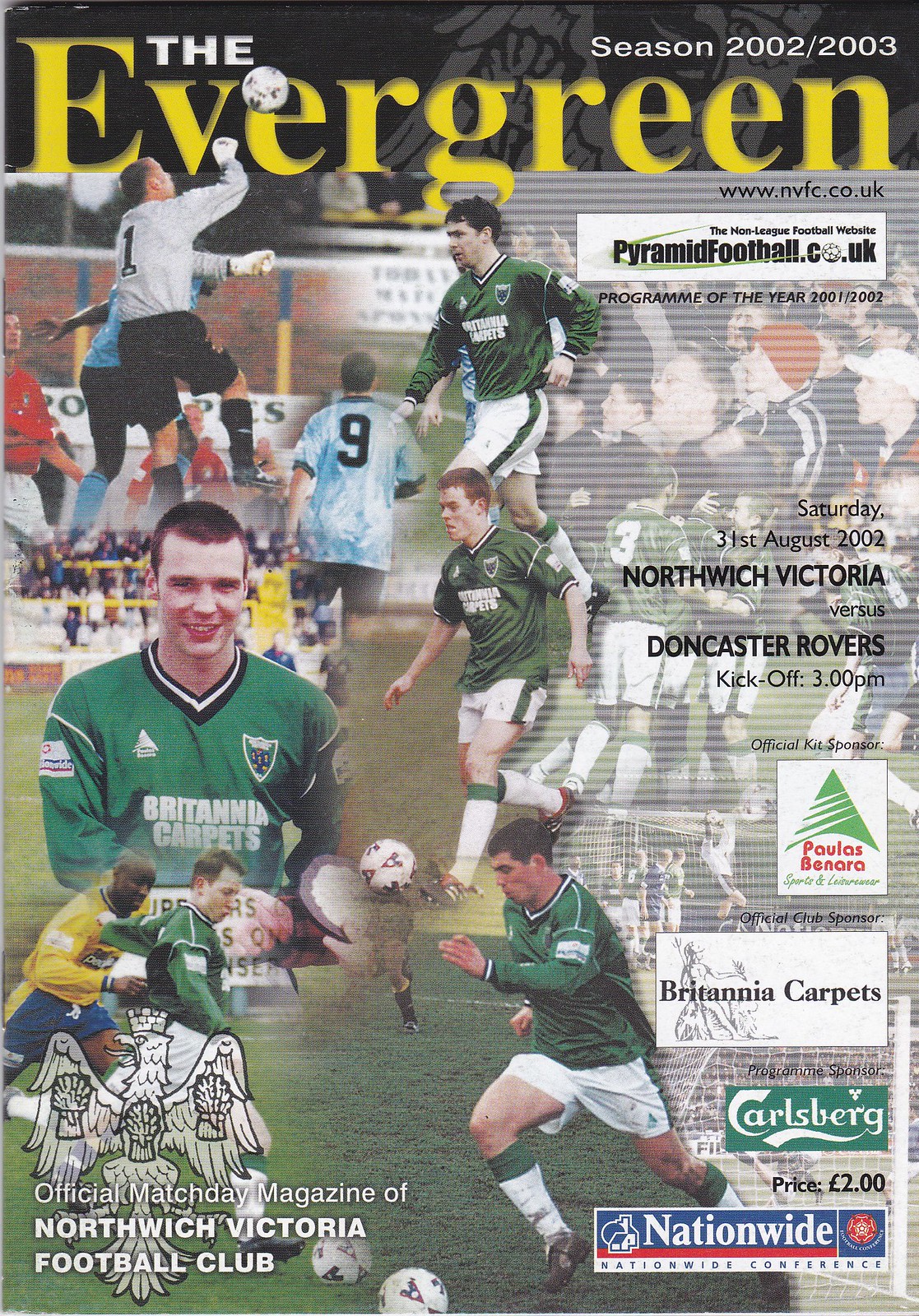This image depicts the cover of the official matchday magazine of Northwich Victoria Football Club, named "The Evergreen." The title "Evergreen" is prominently displayed in bold, Serif font with a yellow color against a black background, accompanied by a detail of a two-dimensional screaming eagle illustration. At the top right corner, the magazine dates the season as "2002 to 2003."

Numerous images of soccer players in action, wearing green jerseys and white shorts with green stripes, are seen crossfading into one another, capturing dynamic moments like jumping for balls and running. The bottom left corner of the cover explicitly notes it is the official matchday magazine. Adjacent to this text is the match information: "Saturday 31st August 2002, Northwich Victoria versus Doncaster Rovers, Kickoff is 3 p.m.," along with confirmation of the official sponsor, Paulus Benaro.

Additionally, the right side of the cover features several logos and web addresses, including one for the non-league football website, pyramidfootball.co.uk.